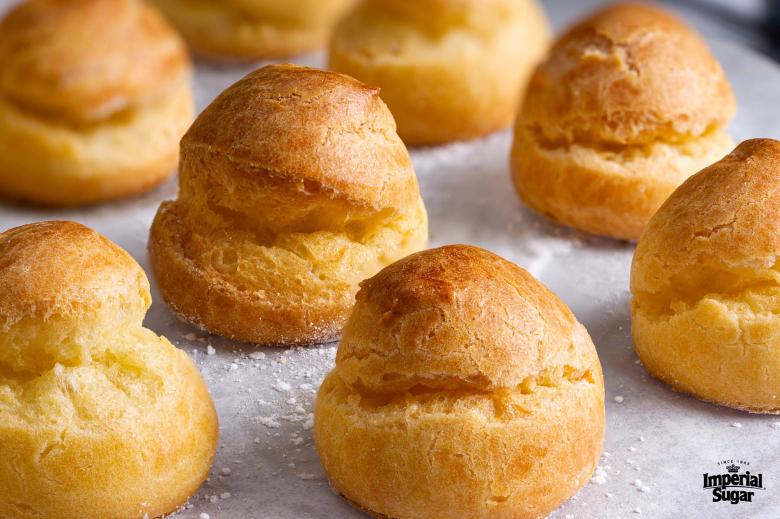Golden-brown and glistening slightly, a collection of freshly baked puff pastry round shells rests on a white parchment-lined baking sheet. Their tops have a delightful sheen, hinting at the buttery goodness within, while a light dusting of flour underneath adds a touch of rustic charm. These airy, fluffy pastries are primed for transformation into delectable cream puffs. Notably, "Imperial Sugar" is printed in the bottom right-hand corner, possibly hinting at the source of the featured recipe or the ingredients used.